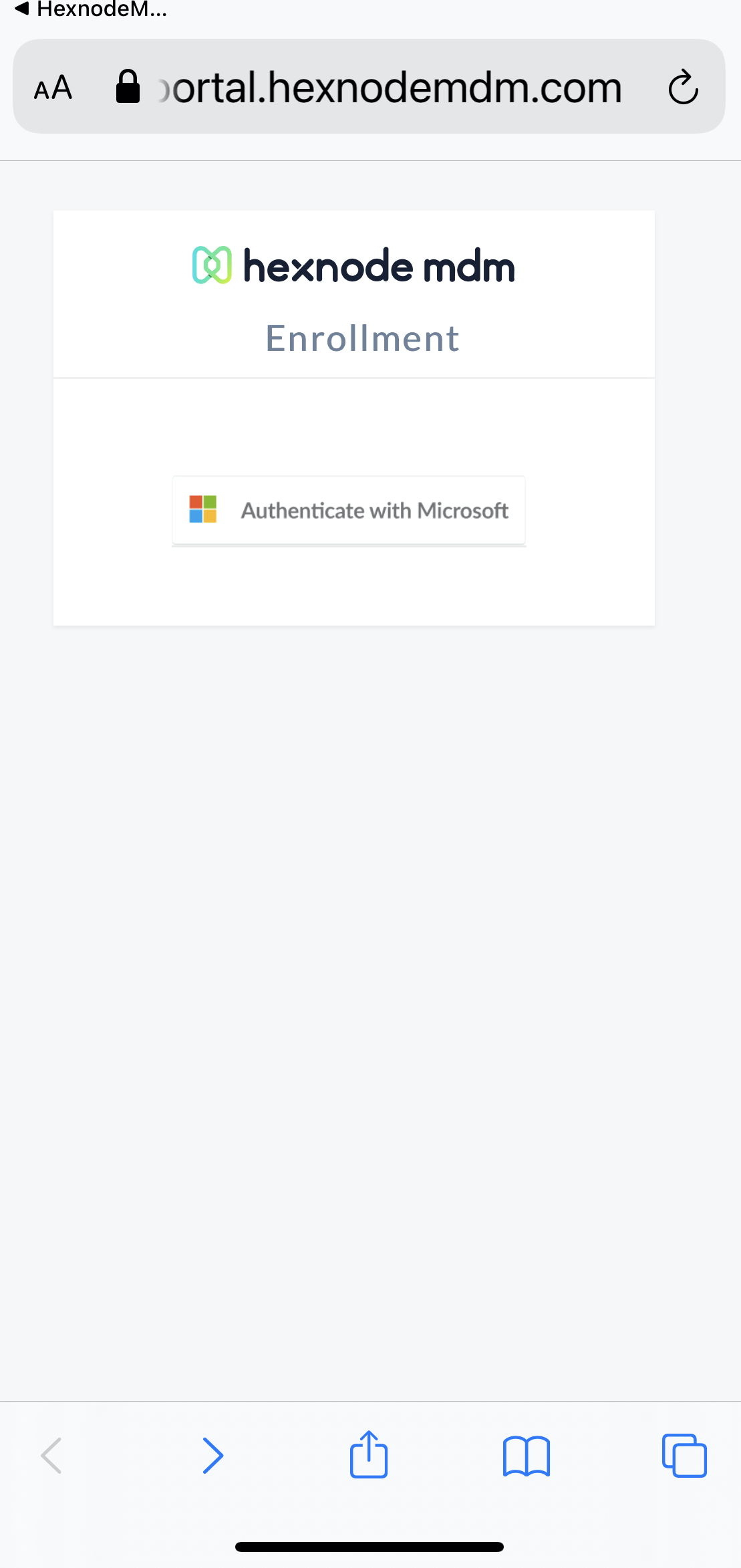This image depicts a smartphone screen showing the website portal.hexnodemdm.com. At the very top of the screen, within the browser's address bar, is the URL "portal.hexnodemdm.com" along with a small padlock icon indicating a secure connection. To the left of the URL is a back arrow button and the beginning of a partially visible web page title, "hexnodem.dot". Below the address bar, the Hexnode MDM logo is positioned on the left side, followed by the word "Enrollment." Beneath this section, there is a horizontal line separating the top part of the page from the next section. Underneath, there is an option to "Authenticate with Microsoft," accompanied by the Microsoft logo positioned to the left of the text.

At the bottom of the screen, typical smartphone browser navigation elements are visible, including a black line. From left to right, these include a left-facing arrow, a right-facing arrow, a download icon, an open book icon, and a tab management icon displaying two overlapping squares. The majority of the middle portion of the screen is predominantly white, signifying either loading content or an empty webpage section.